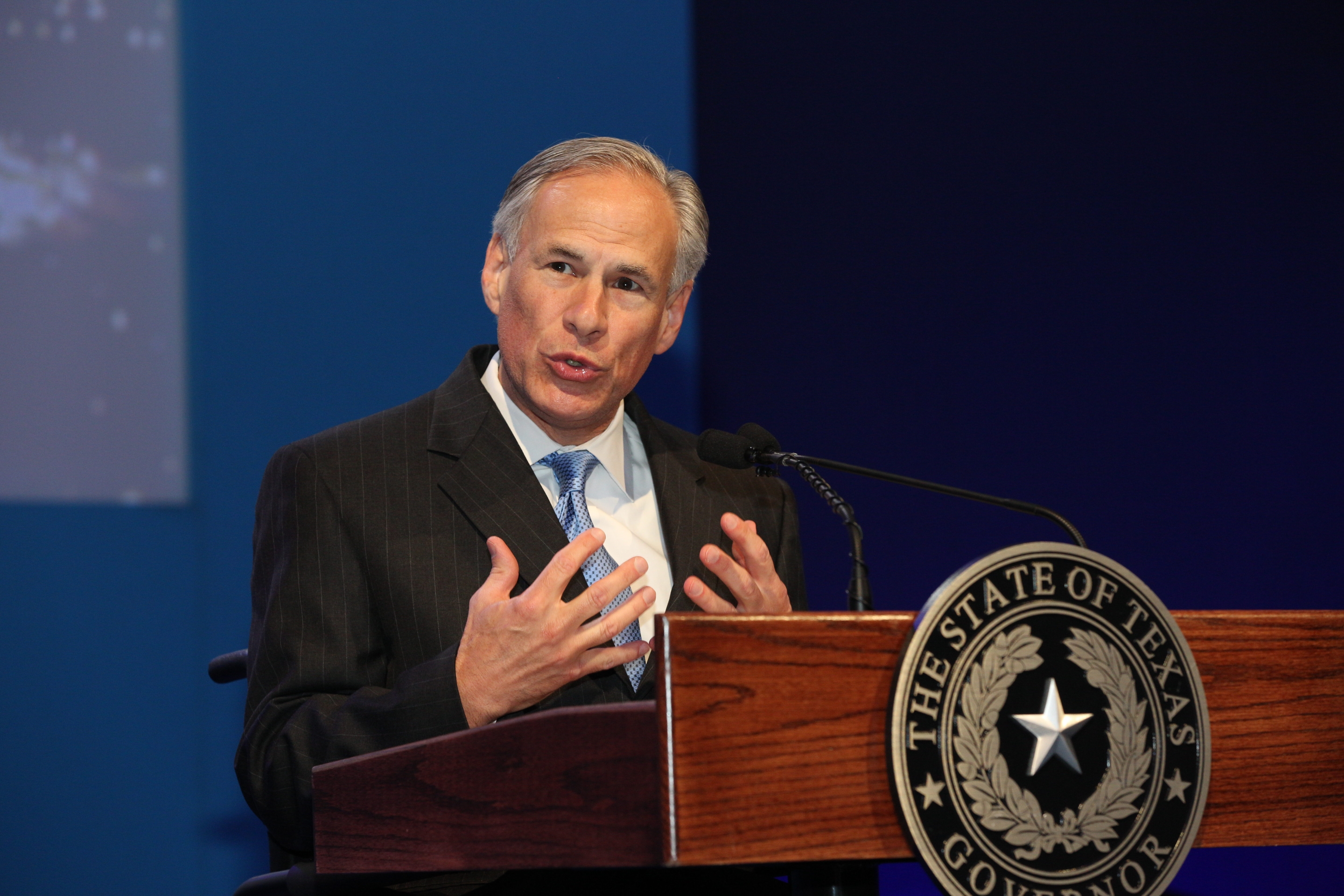The image depicts a distinguished man, presumably the governor of Texas, delivering a speech. He stands confidently behind a brown podium, which features an inscription that reads "The State of Texas" with a prominent star emblem beneath it. The background is comprised of varying shades of blue, with darker tones on the right side gradually transitioning to lighter hues on the left, all of which are softly blurred without any text. The governor is dressed in a well-fitted black suit, complemented by a white shirt and a patterned sky-blue tie. He has grey hair, and his hands are gesturing expressively as he speaks, adding emphasis to his address.